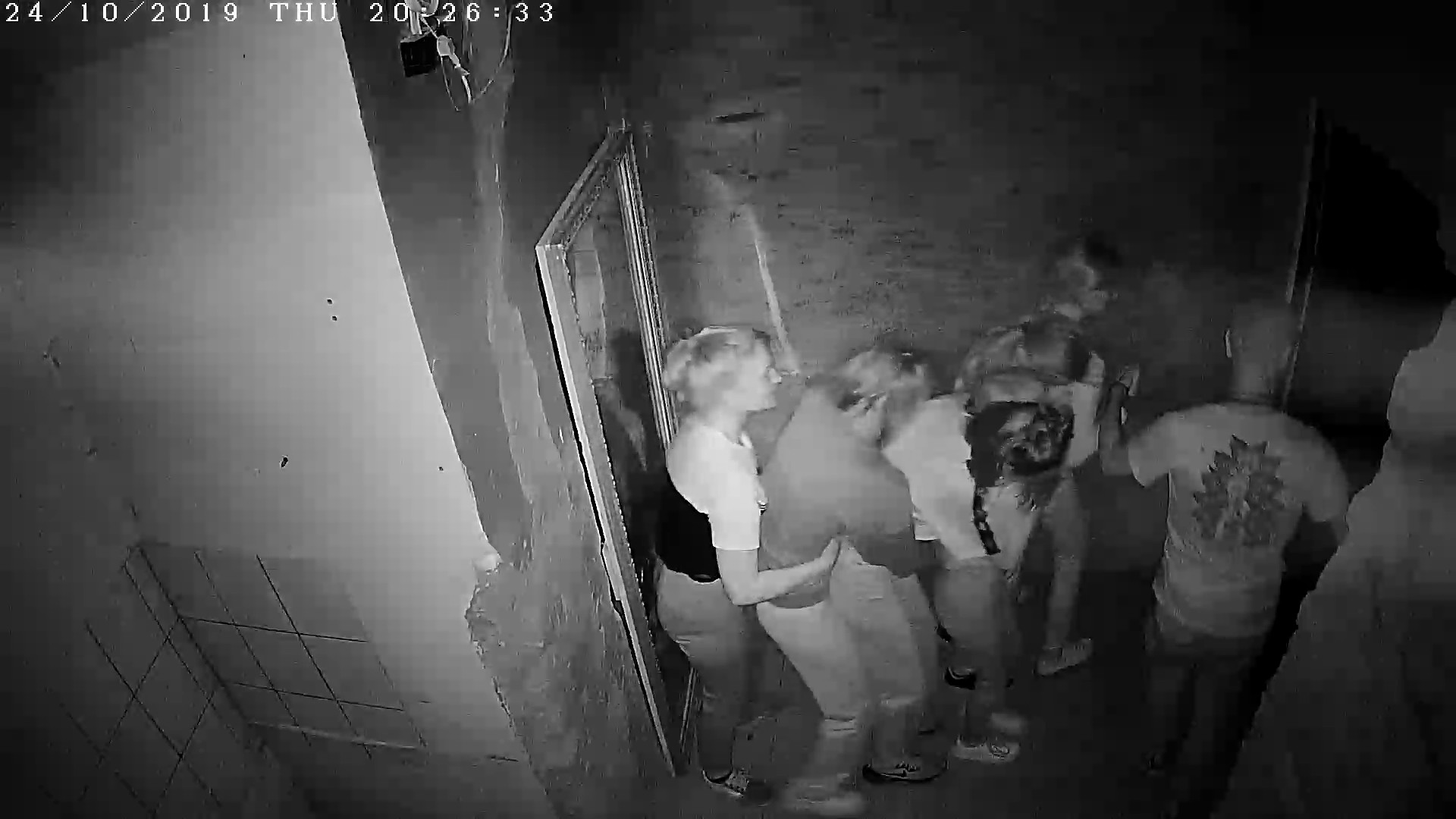This black-and-white photograph, captured by a security camera on October 24, 2019, at 8:26:33 PM, depicts a potentially eerie scene. The image, dark and somewhat blurry, shows a group of six people, possibly teenagers, in what appears to be an unfinished or decrepit interior space with rough, peeling walls and a brick section. The photograph is taken from a high, corner perspective, looking down on the subjects.

The people are huddled closely together in a line, holding each other by the waist, suggesting a haunted house or an escape room scenario. They have just walked through a doorway and are moving towards another dark area. One person, a man, stands slightly apart to the right, wearing a white t-shirt with a pattern on the back, and he is bald. The others, three to five women and possibly two men, are dressed casually, mostly in jeans. The scene is further marked by the time and date stamp in the top left corner along with the European date format (24-10-2019) further underscoring the moment captured in this unsettling yet intriguing snapshot.